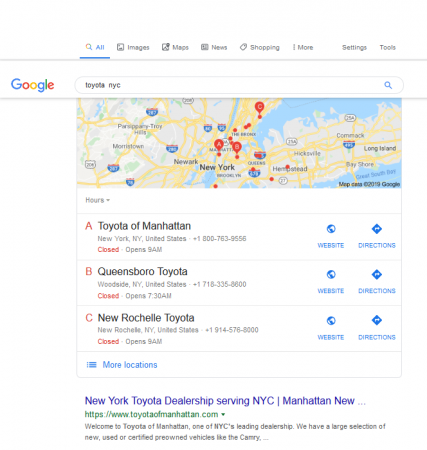The screenshot captures a Google search results page. At the top, multiple tabs are visible, including "All," which is highlighted with a blue underline, followed by "Images," "Maps," "News," "Shopping," "More," "Settings," and "Tools." Beneath this row of tabs is a pale gray horizontal line.

On the left side of the page is the Google logo beside a search bar containing the query "Toyota NYC" in black type. A blue magnifying glass icon is positioned on the far right of the search bar. 

Below the search bar is a narrow rectangular map of New York City, displaying three pins labeled A, B, and C. These correspond to "Toyota of Manhattan," "Queensborough Toyota," and "Rochelle Toyota," respectively, all marked as closed. Each location has accompanying icons for "Website" and "Directions."

At the bottom, in purple type, the text reads "New York Toyota Dealership serving NYC," followed by a green web address. Below this, in black type, is the text: "Welcome to Toyota of Manhattan, one of New York City's leading dealerships. We have a large selection of new, used, or certified pre-owned vehicles like the Camry."